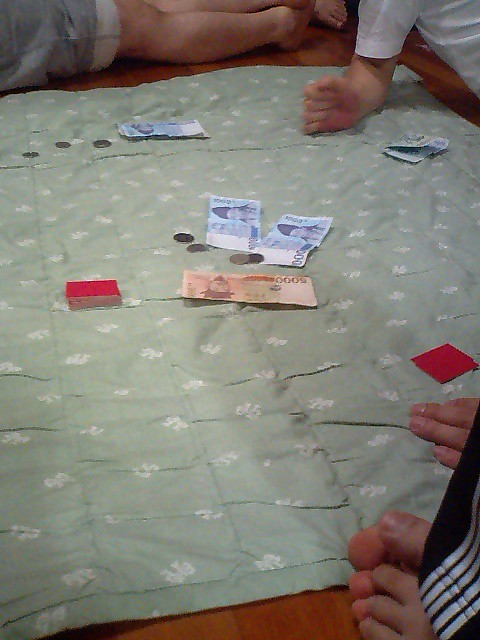The image showcases a green blanket with a white floral pattern spread across a brown wooden floor, possibly hardwood or plank flooring. Scattered on the blanket, several silver coins and multiple foreign currency bills are visible—three are blue paper bills and one is an orange or red bill, the latter featuring the face of an ancient Asian man, possibly Chinese or Korean. On both the left and right sides of the blanket, there are stacks of red cards, suggesting a game in progress, perhaps involving monetary bets. 

In addition to the objects, several people are partially visible within the scene. In the upper right corner, a person wearing a backpack with white stripes is showing their toes. Another individual lies across the floor, wearing shorts and a black-and-white striped garment, and only their legs are visible in the image. Furthermore, a child's arm, donned in a short sleeve white t-shirt, rests on the blanket, and a left hand with visible fingers and pinky is also seen. The overall setting hints at a family or group activity winding down for the night, possibly playing a game involving money.